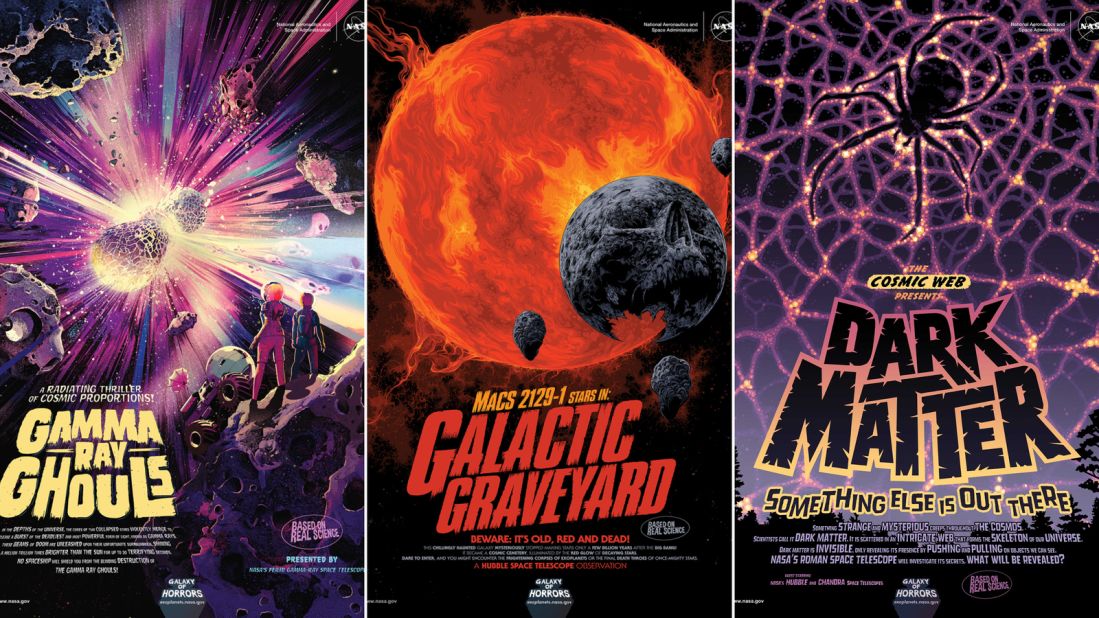This horizontally rectangular full-color image is composed of three vertically rectangular segments, each separated by a thin white line, resembling old movie posters from cheesy horror films. On the left, "Gamma Ray Ghouls" is depicted with vibrant rays of blue, yellow, and purple amid a space setting of flying rocks and cartoon characters standing on a meteor. The central image, titled "Galactic Graveyard," features a large, fiery red star surrounded by asteroids and fragmented planets, with the additional text "Max 2129-1 stars in Galactic Graveyard." The rightmost segment, "The Cosmic Web Presents Dark Matter: Something Else is Out There," showcases a glowing gold and purple spider web with a prominently outlined, luminescent black spider.